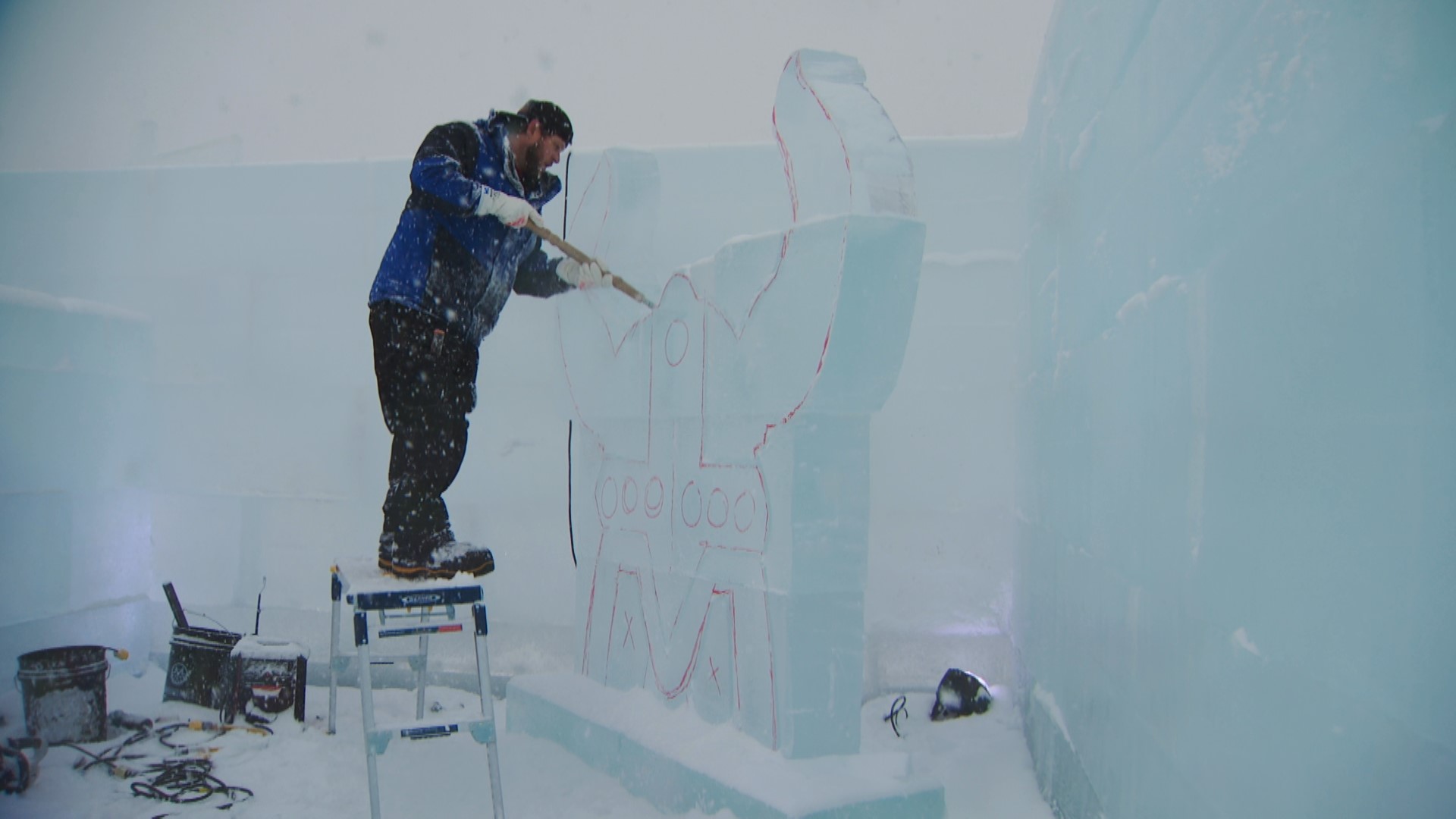This photograph captures an ice sculptor intensely focused on his craft, standing on a blue, three-step stool with metal legs. The man, dressed in a backward black baseball cap, black beard, dark pants, large boots, and a dark blue parka with black stripes, is engaged in the intricate art of ice carving. He holds a long sculpting tool, possibly a pick, and is meticulously working on an ice sculpture in the shape of a crown with Viking helmet-like features. The crown is detailed with large horns on either side, a cylindrical joiner at the top, and a band at the bottom, resembling an upside-down T, topped with a wavy M with cut-open areas marked as Xs. Behind him, there are multiple buckets, one of which contains another tool sticking out, along with wiring essential for his sculpting process. He is surrounded by massive, towering ice walls, which hint at the possibility of the setting being an elaborate ice maze or igloo. The ice he works on and the surrounding structures exhibit a striking blend of white and cyan accents.